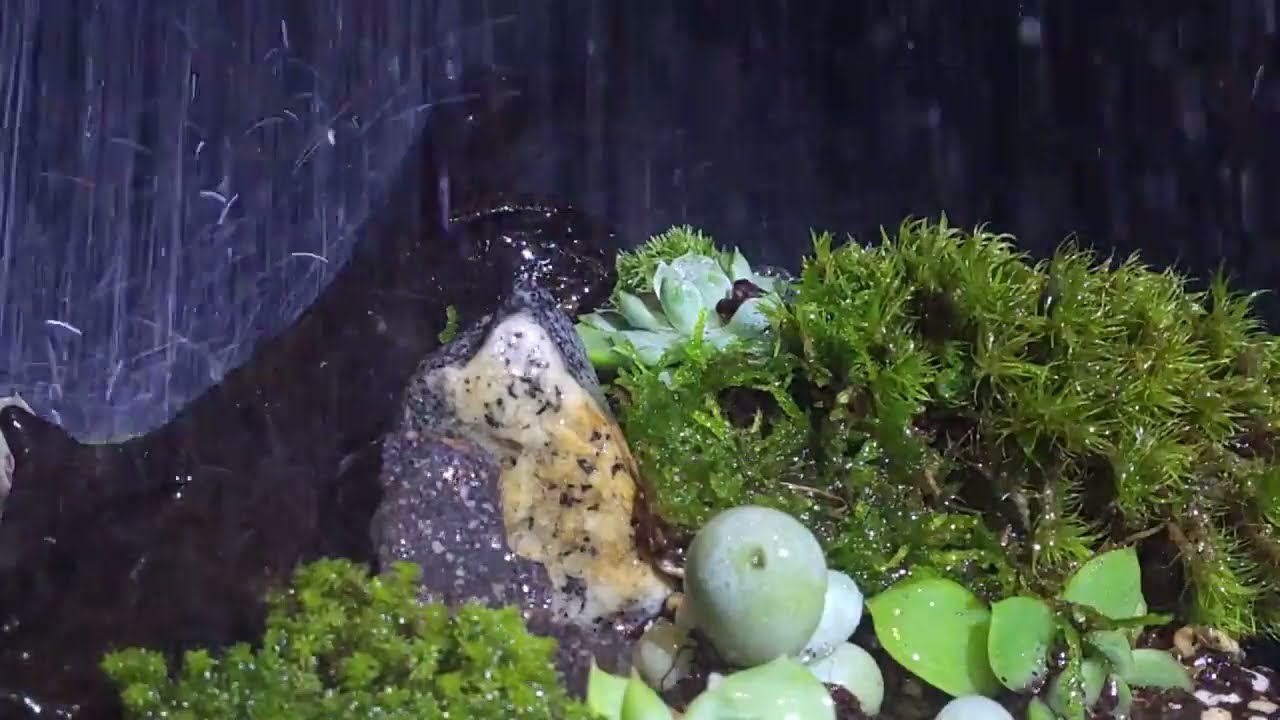The photograph captures a lush, rain-drenched natural scene that appears to be either an outdoor setting or a well-designed indoor aquarium. Dominated by a horizontally rectangular frame, the image features various elements obscured by a downpour, which produces pronounced streaks as water cascades down and splashes off rocks, creating a dynamic backdrop.

In the foreground, a rich array of green, white, and mossy plants flourish. This includes distinct succulents with round formations and little leaf petals that add texture and color to the scene. Among the greenery, a gray rock with a white center and black speckles stands out, flanked by a log on the left. Additionally, there's a noticeable grassy reef area that arches like a hill, contributing to the layered composition of the shot.

The right side of the image remains relatively clear and dry compared to the rest, emphasizing the vivid wetness of the central and left portions. The backdrop, which appears black at first glance, is streaked with rain lines suggesting heavy rainfall. This relentless downpour creates a dramatic visual effect, with water slamming off the rocks and causing a backsplash and spray that enlivens the entire scene.